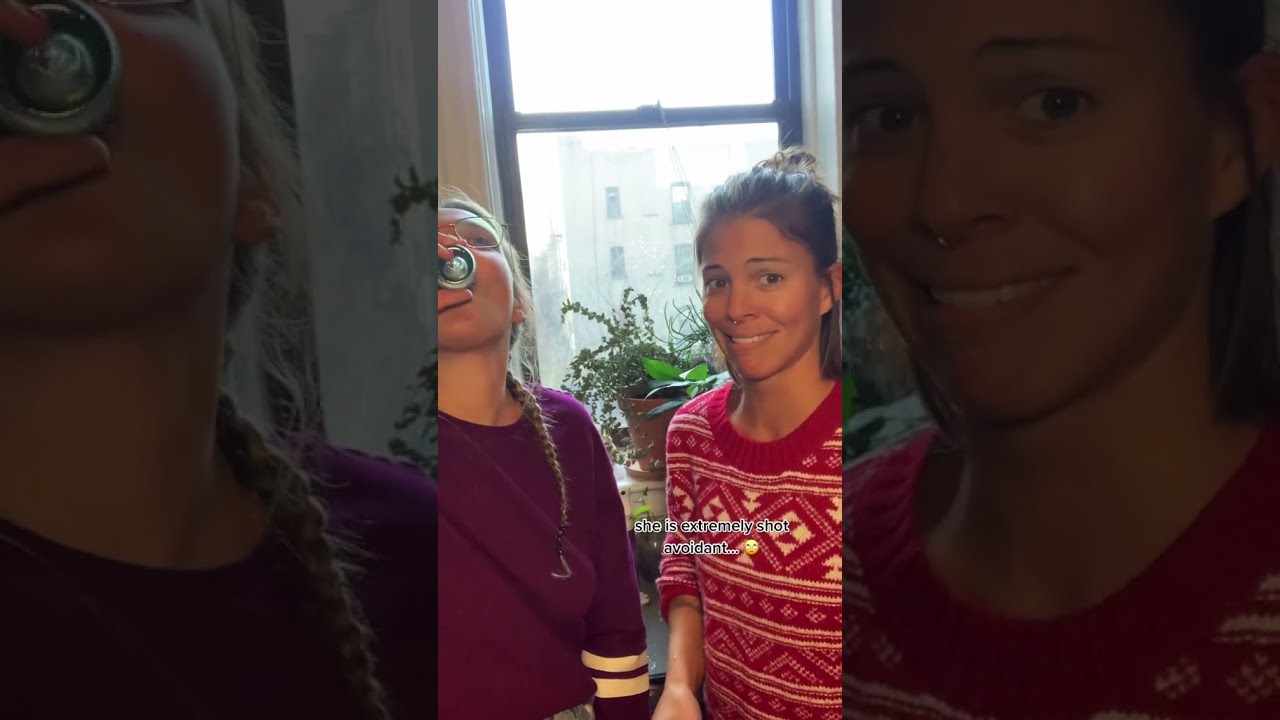The image depicts a photograph, likely a screenshot from an Instagram Story or Reel, taken inside a brightly lit apartment. The scene features two young women, possibly in their late teens to early 20s, standing in front of a window. The woman on the left is wearing a purple shirt with yellow bands on the sleeves. She has her brown hair styled in a braid draped over her shoulder and is seen drinking from what appears to be a shot glass, her glasses slightly reflecting the light. The woman on the right is donning a red sweater with white patterns and has her brown hair tied up in a bun. She also sports a nose ring and appears to be smiling nervously. Superimposed black text in front of her reads, "She is extremely shot avoidant." Behind them, a window reveals a bright exterior, with another building visible in the distance. A potted plant in a terracotta pot is perched on a small stand in the background, adding a touch of greenery to the setting.